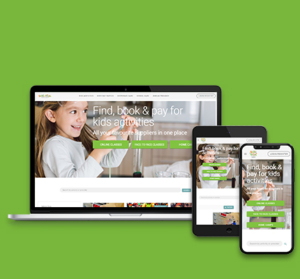Against a somewhat bright olive green backdrop stands a desktop monitor. To the right of the monitor, a tablet is propped up, slightly angled against it. Atop the tablet, a cell phone is similarly leaned, positioned to create a vertical alignment of the devices. Despite zooming out, the text on the screens remains mostly unreadable. However, a portion of a keyboard is visible below the monitor. Each device displays the same image, though the layout varies slightly on the cell phone due to its vertical orientation.

The visible website header showcases a little girl with long brown hair, dressed in a cute gray shirt, holding up an object. The partially readable text beside her suggests that the site is related to children's activities and education, with phrases like "find book and pay for kids activities." Completing the website's interface, there are options for typing in searches and exploring different choices, indicating a user-friendly experience tailored for young learners and their guardians.